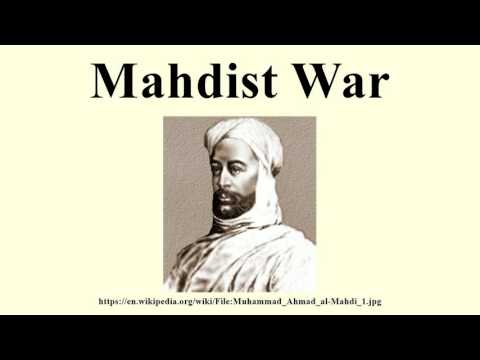The image is formatted like a PowerPoint slide with thick black bands at the top and bottom, creating a movie-like effect. The central background is a pale yellow. In the middle, there's a historical black-and-white photograph of Muhammad Ahmad al-Mahdi, dressed in traditional Middle Eastern attire. He is facing slightly to the left, showcasing his close-cropped beard, angular nose, and his head wrapped in a white turban that extends under his chin. The background of his portrait is a muted brown. Above his picture, the text "Mahdist War" is centered in black, and below the picture, there's a small, centered black text providing a URL: https://en.wikipedia.org/wiki/File:Muhammad_Ahmad_al-Mahdi1.jpg. The overall composition gives off a vintage, scholarly presentation style, emphasizing historical context through subdued colors and clear labeling.